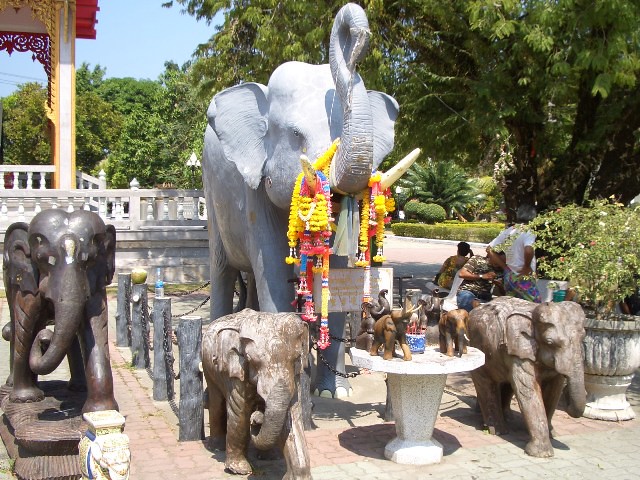The photograph depicts a collection of detailed stone elephant statues situated in what appears to be a park or temple grounds. Dominating the scene is a large, grayish elephant statue adorned with colorful, decorative flower garlands hanging from its tusks. This prominent statue stands with its trunk raised, possibly suggesting the flow of water. Surrounding this main figure are several smaller elephant statues, which are predominantly brown in color, with some faded due to weathering. These smaller statues have their trunks pointing downward and are arranged around a flat-top pedestal table that holds additional tiny elephant statues.

In the background, the scene is framed by lush greenery, including trees, bushes, and a large planter with a plant, hinting at a verdant, almost tropical environment. Chains link gray posts, forming a barrier around the statues. To the left, another slightly larger brown elephant statue is perched on a pedestal, with further small stone figures scattered around. Behind the statues, there are more signs of human presence, like people, white railings, and possibly a road. To the right, a building with a yellow roof and red and yellow molding suggests the nearby structure is part of the temple or park setting. The combined scenery with its statues, greenery, and architectural elements creates a rich, culturally infused tableau.